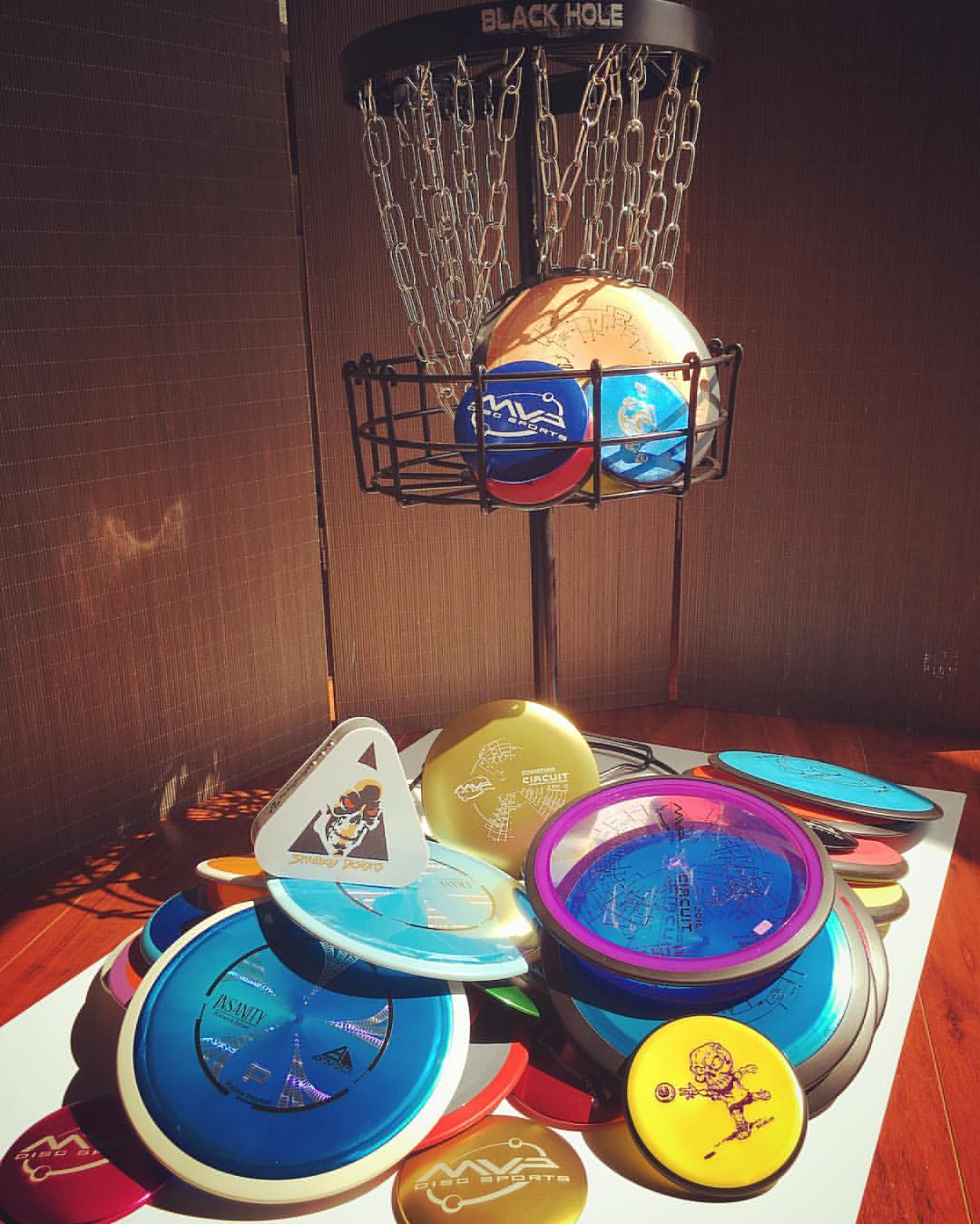The image features an arrangement of various disc-shaped items, predominantly frisbees, placed on a reddish wood table with a white paper mat or cloth. At the center top, there's a black metal disc golf basket labeled "Black Hole." This basket includes a cylindrical top with silver chains hanging down and a wire basket beneath, attached to a rod extending downward. The basket serves as a target for the frisbees. Inside the basket are several frisbees, including a large orange one and smaller ones in dark blue, light blue, and red. Scattered across the table are more frisbees, described in a variety of colors and sizes: blue with silver rims, blue with white rims, light blue, yellow, gold, red, a tan frisbee, and one with a purple rim featuring a skeleton graphic. There is also a notably triangular disc among them. The setup includes a black backdrop partitioning the view, focusing attention on the frisbees and the basket.